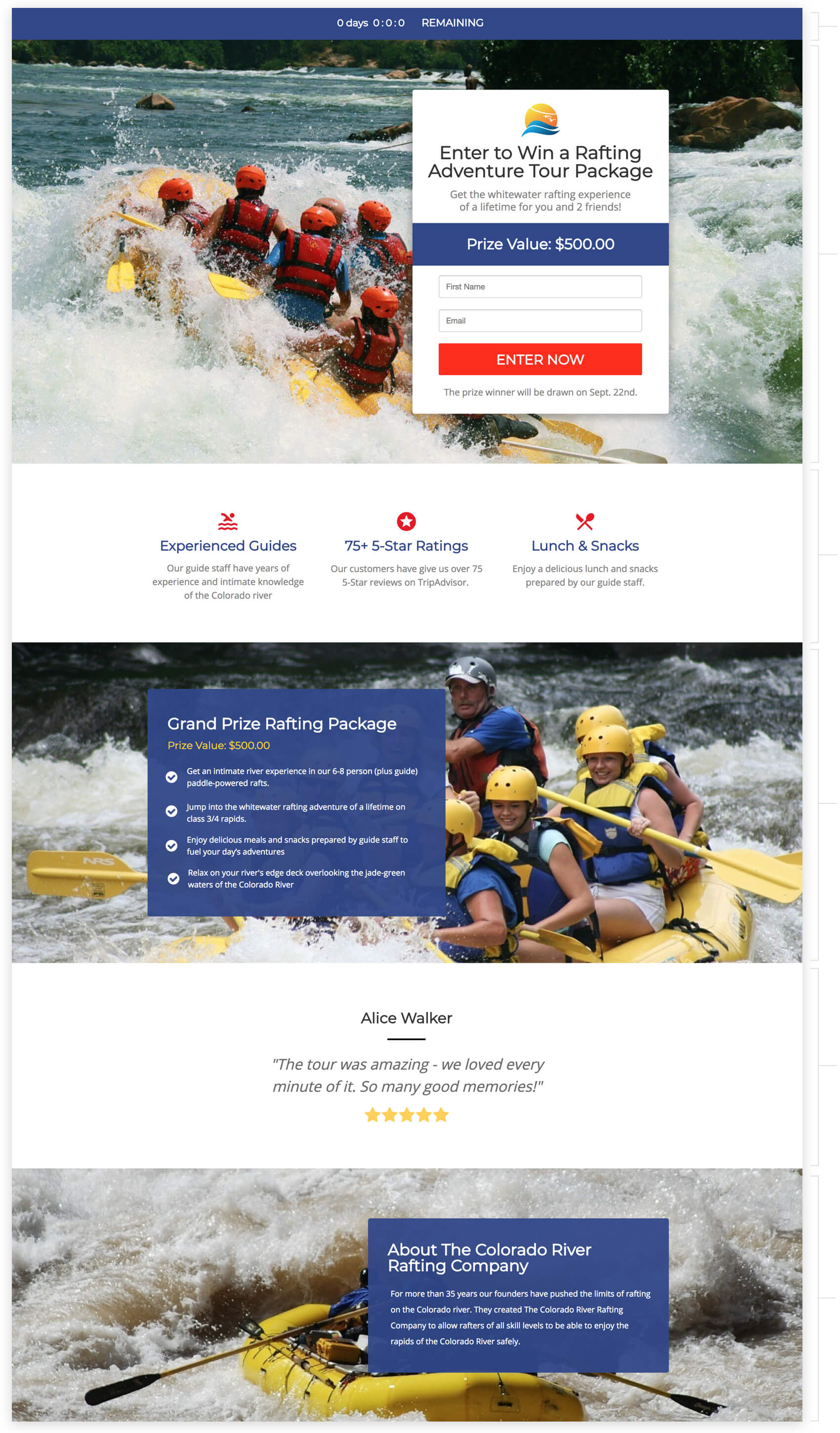A smartphone screenshot captures a whitewater rafting advertisement presented in a triptych layout. At the top, a bold banner declares "0 Days, 0 Hours, 0 Minutes Remaining," indicating the urgency of an ongoing promotion. The first image in the sequence features a raft maneuvering through turbulent waters, filled with seven visible adventurers (although partially obscured by a pop-up). The pop-up overlay invites viewers to "Enter to Win a Rafting Adventure Tour Package," valued at $500. This overlay includes fields for entering a name and email address, along with an "Enter Now" button. Below this, a highlighted section emphasizes the quality of the experience, boasting "Experienced Guides," "75+ Five-Star Ratings," and the inclusion of "Lunch and Snacks."

The second photograph showcases another raft navigating the river, with six participants onboard. This image also has a pop-up reiterating the grand prize's value at $500. Further down, a testimonial in a white space captures a glowing review from Alice Walker: "The tour was amazing, we loved every minute of it, so many good memories!" She awards the experience a full five-star rating.

The third and final image presents a raft amidst the rapids, steered by one visible person with two oars extending into the water. An overlay on this image provides information about the Colorado River Rafting Company, tying all elements of the advertisement together.